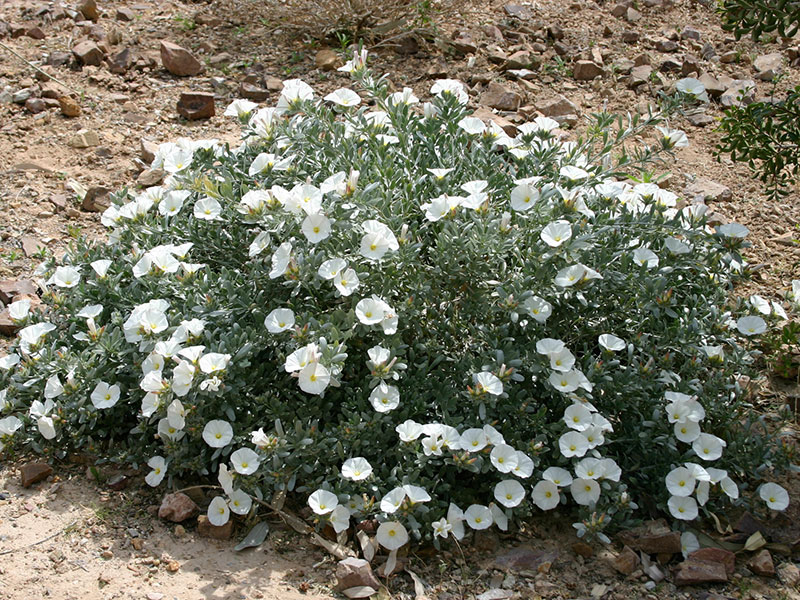In the image, a sprawling, low-to-the-ground bush is adorned with an abundance of small, white flowers resembling morning glories. The flowers are in full bloom, each featuring a prominent yellow center. The bush's numerous tiny green leaves contribute to its shrubby, expansive appearance. It stands out vividly against the predominantly dry, rocky terrain that characterizes the background, which includes several large rocks and pebbles scattered both in front and behind the bush. The only other greenery visible is a small branch in the top right corner of the image, enhancing the stark contrast between the lush bush and the barren, desert-like surroundings.